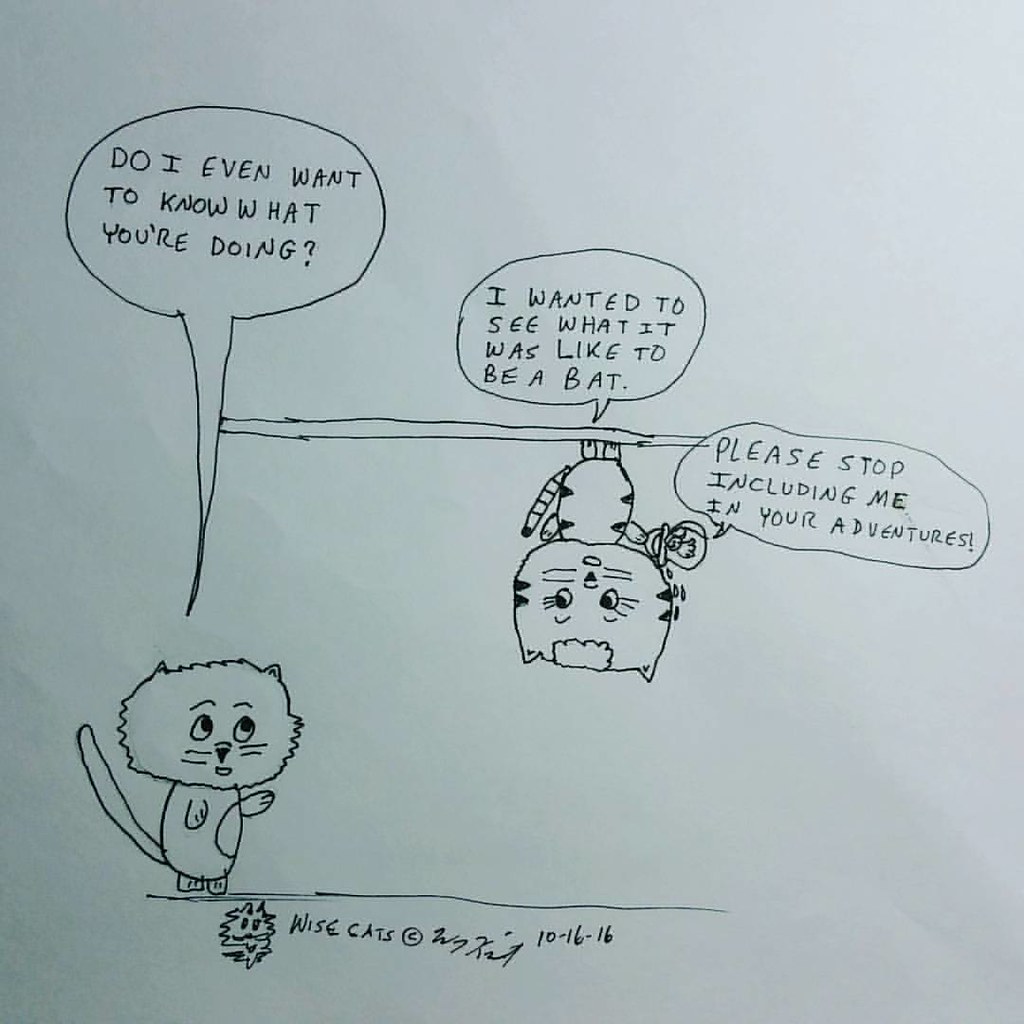This detailed photograph captures a hand-drawn cartoon on what appears to be a slightly gray paper, perhaps due to lighting. The drawing, made entirely in black ink on a white sheet, consists of two anthropomorphic cat characters. 

In the lower-left corner, a cat stands on its hind legs, looking up at a tree branch from which another cat is hanging upside down by its feet. The standing cat has a speech bubble that reads, "Do I even want to know what you're doing?" The hanging cat, looking back down at the ground, has two speech bubbles. The first says, "I wanted to see what it was like to be a bat," while the second, slightly to the right, says, "Please stop including me in your adventures." There also appears to be a small fishbowl with a goldfish near the hanging cat, although it is quite small and hard to distinguish.

Below the scene, at the very bottom of the paper, is the artist's signature "Wisecat" next to a fuzzy cat face drawing, followed by a copyright symbol "C" in a circle and the date "10-16-16." This charming sketch captures a playful and humorous interaction between the two cat characters.